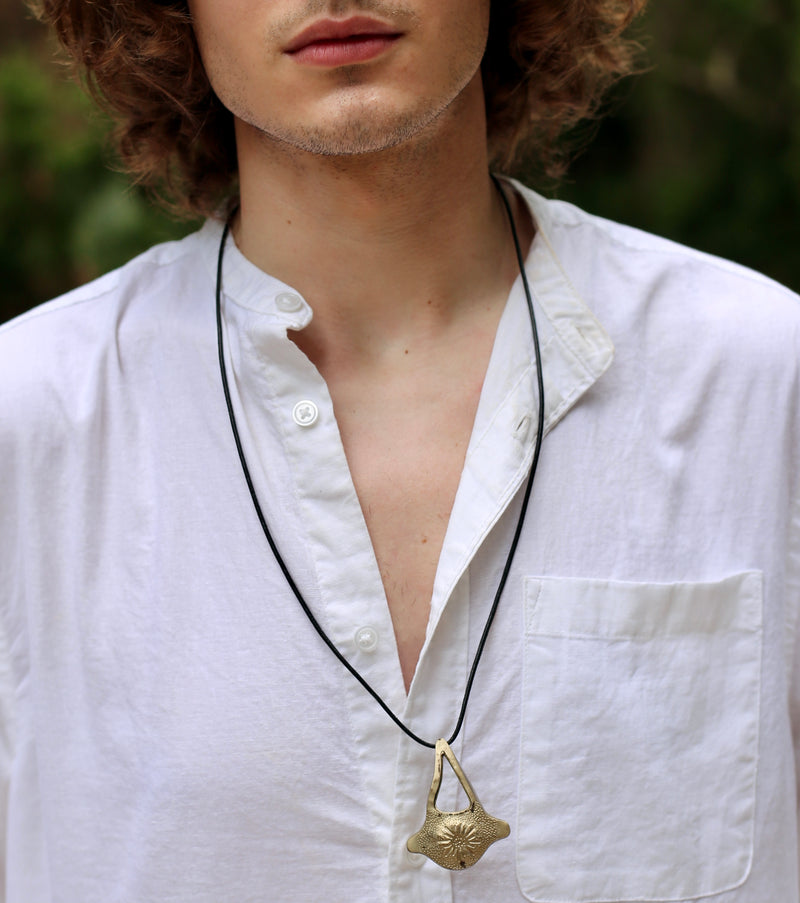A young man with shaggy brown hair and some facial hair visible underneath his chin and on his upper lip is seen in the image, which captures only the lower third of his face. He is wearing a white, loose button-up shirt with the top two or three buttons undone, revealing part of his chest. Attached to his neck by a simple black string necklace is a matte gold pendant shaped like a triangle, featuring an oval embellished figure that protrudes outward, reminiscent of a textured, bowl-like form. The shirt also has a pocket on the right side, which appears to be empty. The background suggests he is outdoors, likely in front of a group of trees, as indicated by the varying shades of green visible behind him.